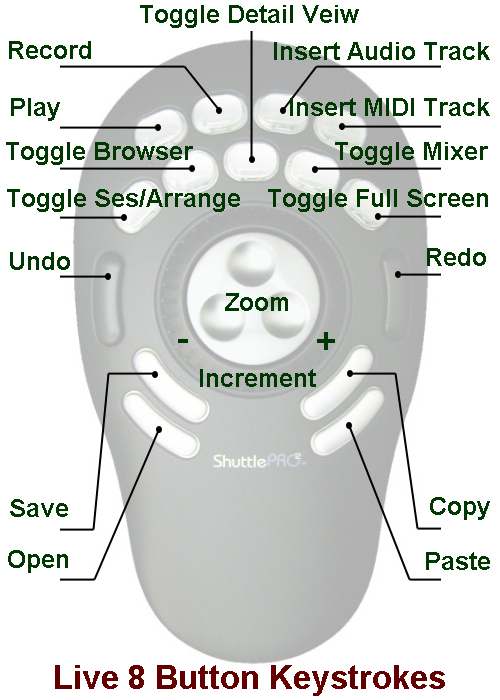The image depicts the detailed mechanics of a computer accessory, identified as a "Shuttle Pro" remote control. The remote is oval-shaped, with a faint illustration in the background, and features an array of buttons, each labeled with specific functions. At the very top are four white buttons, followed by a set of five white buttons below them. Further down is a central circular section with three buttons arranged in a triangular configuration. Flanking this circle to the left and right are gray, jellybean-shaped buttons. Below the central circle are four additional white jellybean-shaped buttons. Each button has a black line extending from it, leading to text that explains its function in detail. The labels include "toggle detail view," "insert audio track," "insert MIDI track," "toggle mixer," "toggle full screen," "redo," "zoom," "increment," "copy," "paste," "open," "save," "undo," "toggle SES arrange," "toggle browser," "play," and "record." At the bottom of the image, highlighted in red, the text reads "Live eight-button keystrokes."